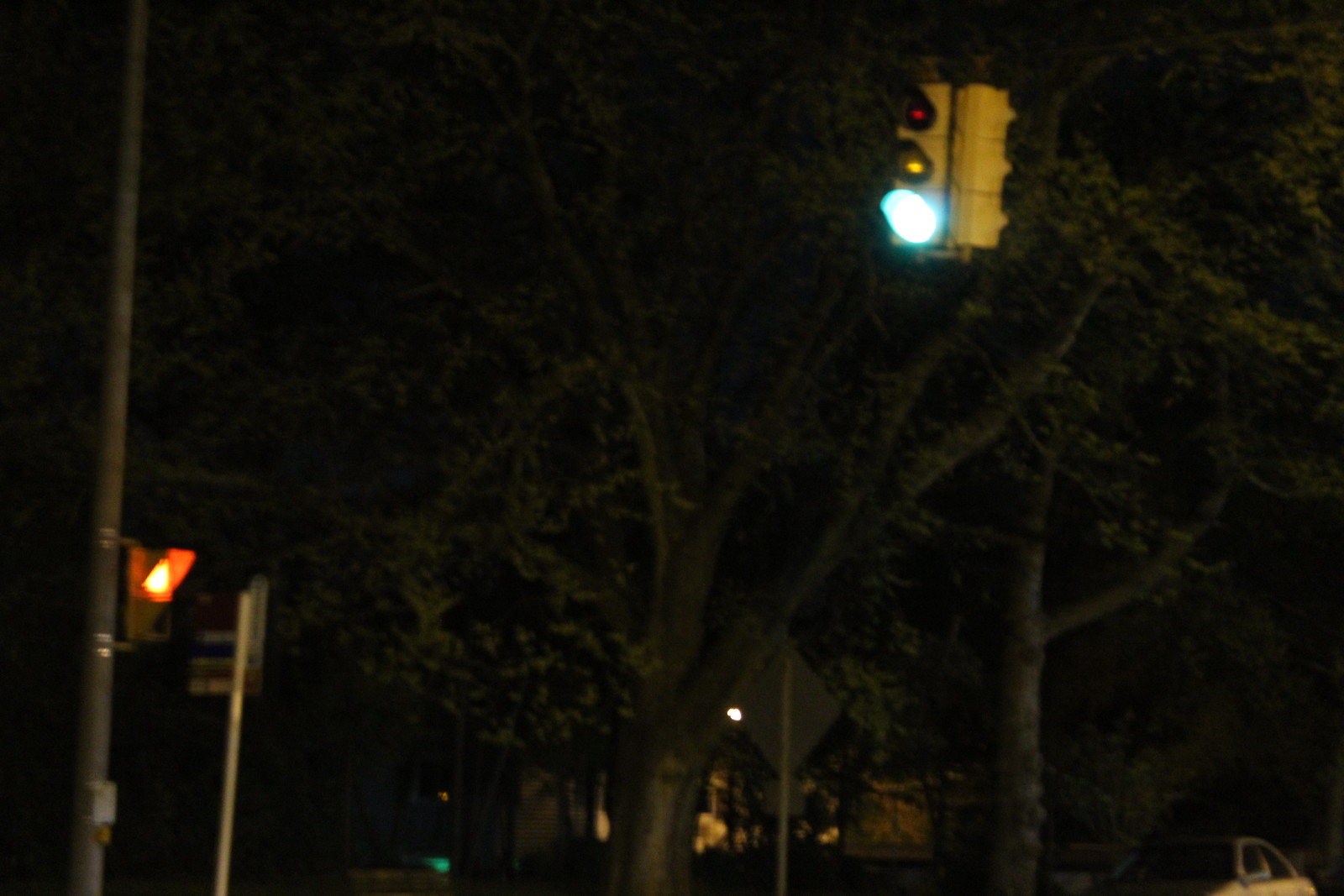This nighttime photograph captures a traffic light prominently featured in the upper portion of the frame, glowing a bright green. The traffic light follows the traditional red-yellow-green format and lacks any additional lights for turns or turn arrows. Suspended by a wire, the traffic light appears to float against a dimly lit backdrop. Despite the darkness, the scene is sufficiently illuminated to reveal medium to large-sized trees in full foliage. Adding to the urban atmosphere, the image includes the rear view of a diamond-shaped street sign and a lamppost situated on the left edge. The lamppost features an illuminated orange "Do Not Walk" signal, contributing to the ambient cityscape.